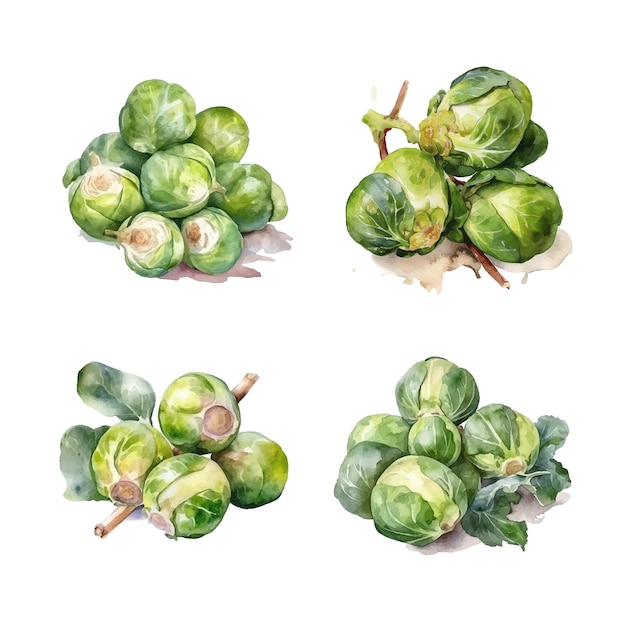This vivid and detailed illustration, set against a clean white background, showcases four distinct clusters of Brussels sprouts in a watercolor-style painting. The Brussels sprouts are depicted in a bright, vibrant shade of green, with peeking darker green leaves and occasional white highlights. Each cluster is arranged in specific positions: one lies in the upper left, another in the upper right, a third in the bottom left, and a fourth in the bottom right, with white space separating them. These small, spherical vegetables feature little brown nubs at their bases where they were picked, adding a touch of mocha color. Some sprouts exhibit a bit of unraveling of their outer leaves, revealing multiple shades from the darker outer leaves to the lighter, fresher inner layers. This highly detailed artwork includes slight drop shadows to enhance the three-dimensional effect and emphasize the detailed textures and colors of the Brussels sprouts.